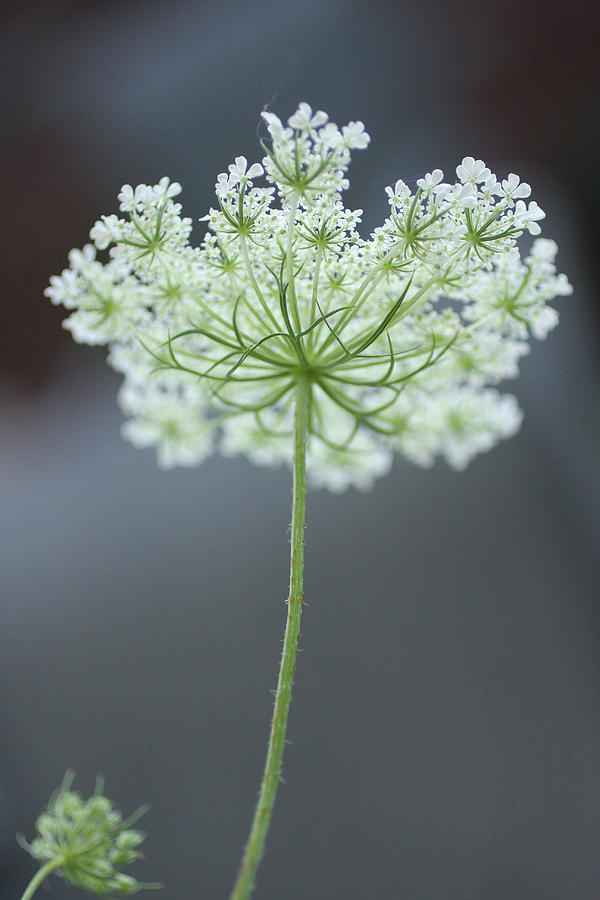The image is a close-up photograph of a delicate white flower with a long green stem, set against a dark gray background. The flower resembles a dandelion, featuring an array of small, tiny white petals that emanate from the stem, creating a shape similar to an umbrella. The flower has a compound structure with pin-like leaves underneath. The bottom part of the image is out of focus, while the top part is clearly defined. There is also a blurred outline of a similar flower in the right corner. The intricate details suggest it could be a wildflower commonly found in the countryside, possibly suitable for use in wedding bouquets or head veils.